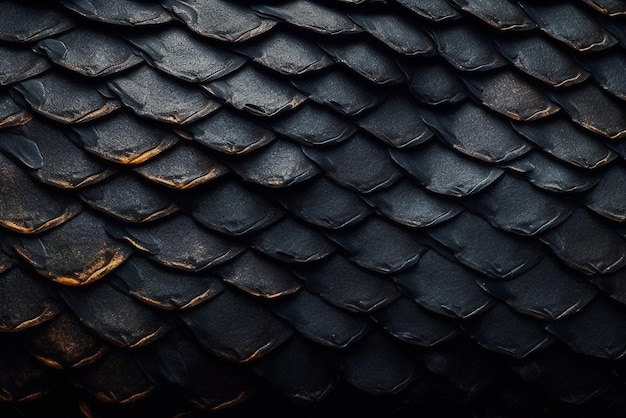This up-close photograph features a dark, textured, and highly detailed surface resembling scales, evoking the tough, reptilian hide of a dragon. The scales, numbering over 150, are arranged in several interconnected rows, appearing blackened with variations of gold trim along their edges. The scales are predominantly black, with a noticeable lighter tint where the light strikes certain areas, particularly on the upper portion and stretching diagonally from the left to the right. The gold trim is more prominent on some scales on the right-hand side and the bottom left corner, suggesting a source of light or fire illuminating parts of the image. The scales vary in size but maintain a uniform, overlapping arrangement, creating a realistic 3D texture. As the image progresses towards the bottom, the scale details become harder to distinguish, fading into a darker, almost night-like appearance. The overall effect is a striking portrayal of a dark scaly surface, rich with intricate detail and textural contrast.